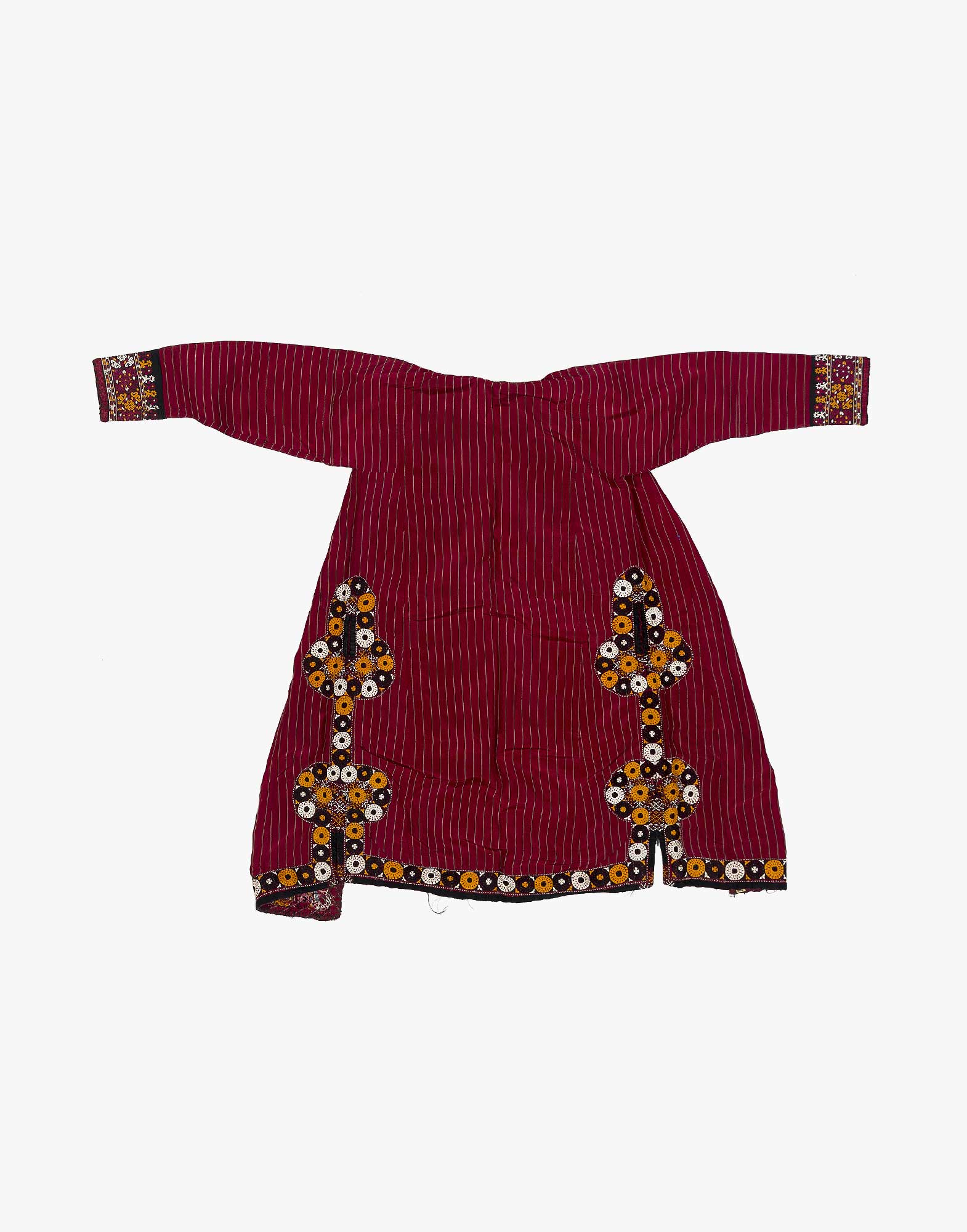This is a photograph of a red garment, either a long blouse or a coat, laid out flat on a white background. The shirt-like top features long sleeves and is decorated with intricate patterns. The fabric showcases thin vertical white stripes and boasts elaborate beadwork along the cuffs and bottom hem. The cuffs of the sleeves are adorned with blue, gold, and red designs, while similar patterns embellish the hemline. Unique sequin details rise up at two points near the sides of the garment, forming vertical lines with bisecting circular patterns in alternating colors of white, black, gold, and brown. The garment is depicted in a T-shaped position with arms outstretched, slightly billowing outwards. The back of the blouse has two slits, each surrounded by the same hem design, adding to the intricacy of this children's clothing piece.